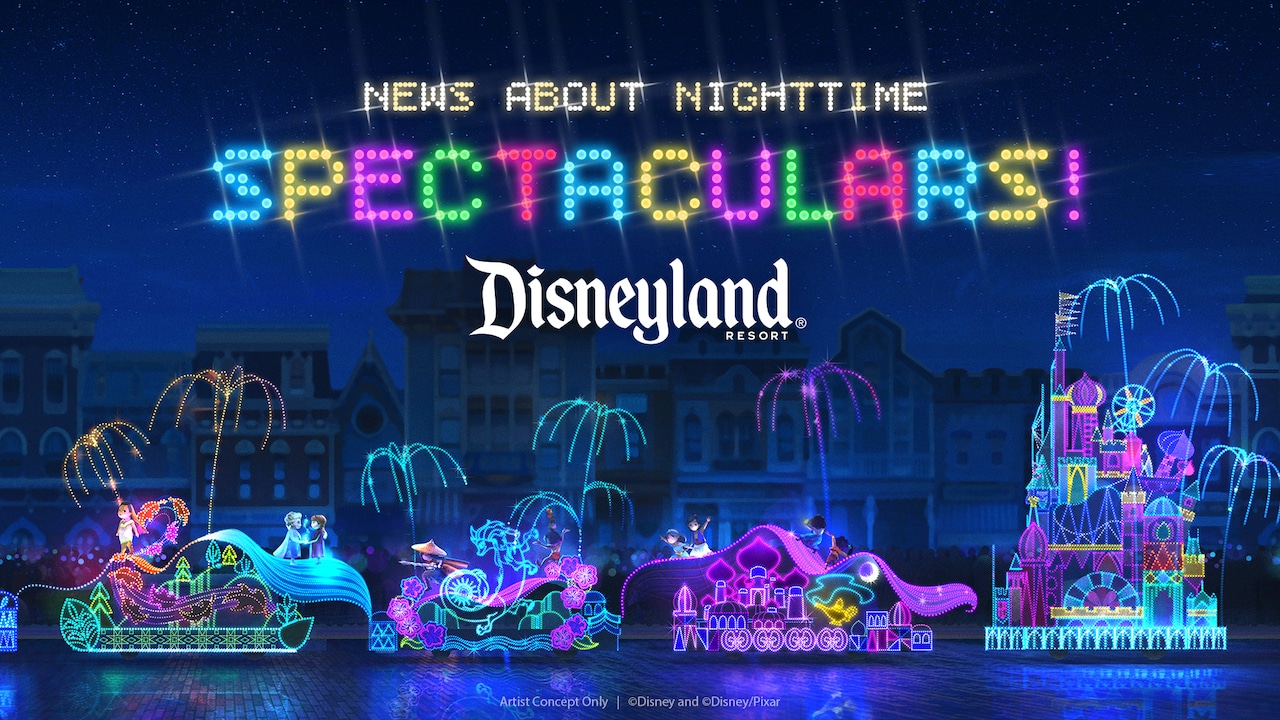This vibrant, colorful advertisement for Disneyland Resort captures the magic of nighttime spectacles with a dark blue backdrop and a riot of neon lights. At the top, glowing in bright white neon, the text announces "News About Nighttime," followed by "Spectaculars" spelled out in alternating neon colors—blue, yellow, pink, green, and red—with a pink exclamation mark for extra flair. Below, in bold white letters, it declares "Disneyland Resort."

The scene beneath this vivid announcement is equally enchanting. A blend of European-style buildings and famous Disney landmarks like roller coasters, the Disney castle, and lively fireworks create a whimsical background that dazzles under the night sky. Palm trees adorned with yellow, turquoise, and purple lights enhance the magical ambiance.

Dominating the foreground, a shimmering body of water reflects the neon lights, making it appear almost purple-blue. Here, a parade of boats trimmed in radiant neon lights float, each representing beloved Disney scenes. One boat resembles a sleigh adorned with candles, possibly featuring Frozen characters; another seems to depict a scene from The Little Mermaid. There’s a boat with a purple theme and what looks like a castle-inspired design. The iconic Ferris wheel and a stylized Disney castle also make an appearance, tying the vibrant, dreamlike photo into a cohesive, enchanting celebration of Disneyland's nighttime extravagance.